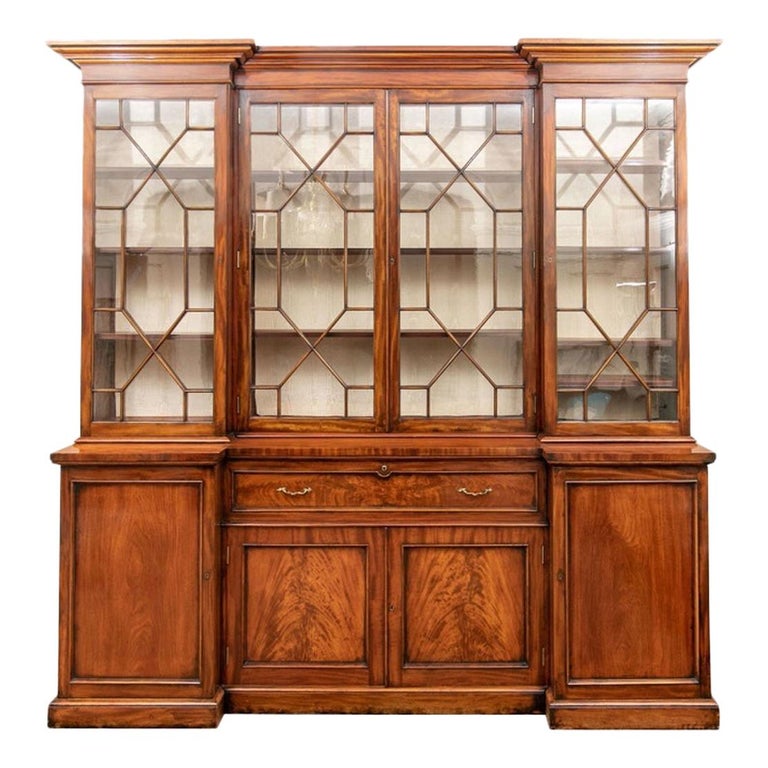This image depicts an elaborate, multi-component China cabinet made of medium-toned, caramel-colored cherry wood. The cabinet features a symmetrical design with a wide central section flanked by two narrower piers. The central portion comprises opposing glass doors elaborately outlined with a brass-lined geometric lead design that opens to reveal a spacious interior. Below the glass doors, a long drawer spans the width of the central section, and beneath this, there are two square, hinged-door cabinets. The side piers also have glass doors with matching geometric designs and storage compartments inside. The entire top of the cabinet is a tall, rectangular glass case with four large, vertical doors, white background contrasts with the brown wood and provides a backdrop for three shelves. The upper part is flat with subtle triangular corners, maintaining the rich, medium wood stain throughout. The cabinet combines both display and storage functionalities, making it a sophisticated focal point for showcasing fine China.